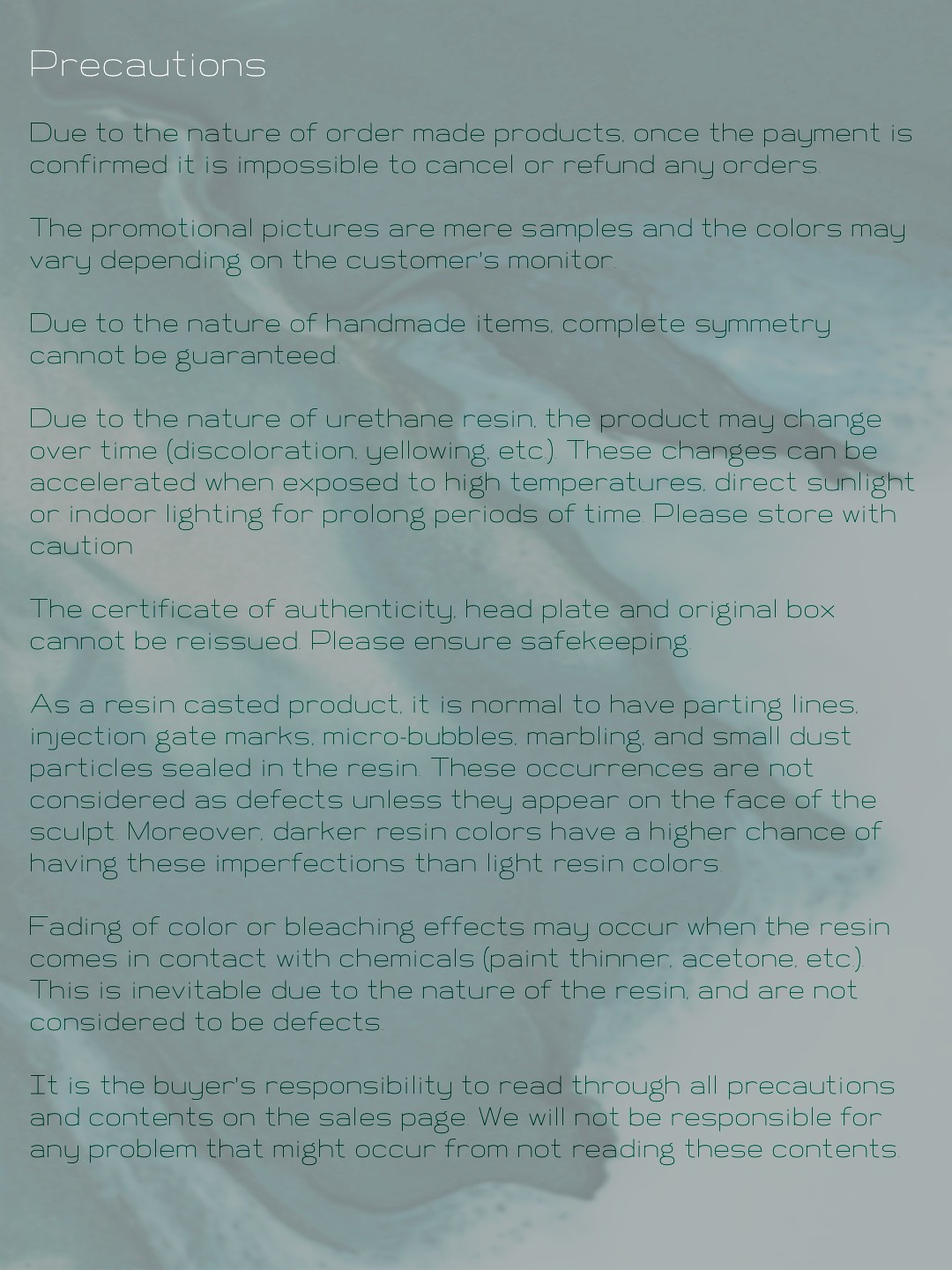The image depicts a full-page advertisement on a piece of paper, closely resembling the dimensions of a standard sheet. The background features a distinct green shade with an intricate design, possibly resembling a dragon or lightning symbol in a pale whitish hue, subtly embedded behind the text. Centered at the top in bold white letters is the title "Precautions". Beneath this title, in darker green text, the page is segmented into eight paragraphs containing vital disclaimers.

The first line of text states, "Due to the nature of order-made products, once the payment is confirmed, it is impossible to cancel or refund any orders." Following this, another notice warns that "the promotional pictures are mere samples, and the colors may vary depending on the customer's monitor." Further disclaimers highlight that "complete symmetry cannot be guaranteed due to the nature of handmade items," and that "products made from urethane resin may change over time." Additional text advises that a "certificate of authenticity, headplate, and original box cannot be reissued," emphasizing the importance of safekeeping.

Overall, the document serves as an exhaustive list of legal disclaimers designed to protect the company against potential customer complaints regarding their products.